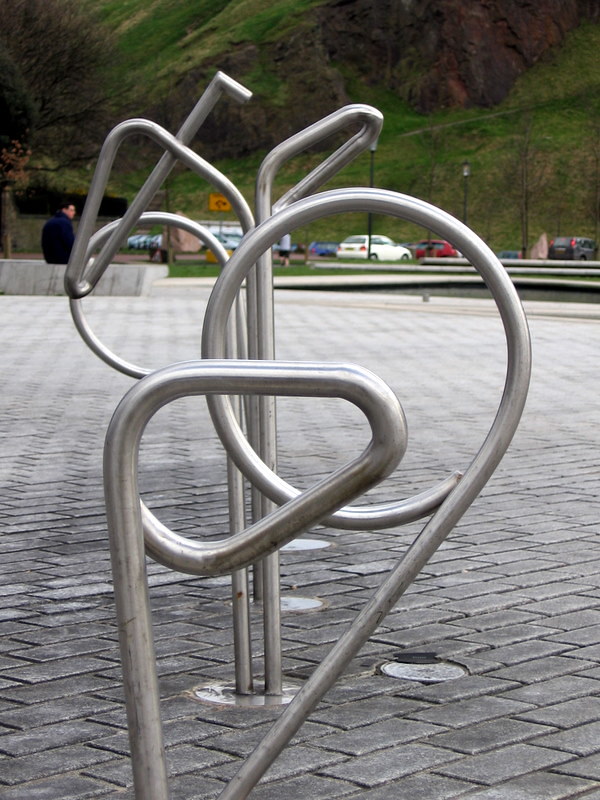The image depicts an outdoor scene centered on a grayish brick walkway that serves as a base for an intricate metal sculpture, which likely functions as a bike rack. The bricks are uniformly rectangular and lead up to the two-thirds mark of the photograph. The metal sculpture consists of multiple interconnected metal posts. Starting just left of center, one pole ascends and curves into a triangular loop, then circles around. Another post extends to the right, forming a large circle behind the triangular structure. Two more metal posts rise in the background; the one on the left makes a leftward loop, while the right post shapes into another triangular form. The sculpture's design resembles components of a bicycle, with the front section evoking a bike seat and the rear resembling bike wheels and handlebars. 

In the upper third of the image, a person sits on a stone bench, which appears to be part of the park where the photograph was taken. Behind this, a mix of parked cars and a large mountain range — painted in shades of red, gray, and brown — stretches across the background. Scattered trees can also be seen amidst this natural backdrop, enhancing the outdoor ambiance. The photograph, oriented vertically, measures approximately six inches tall and four inches wide.